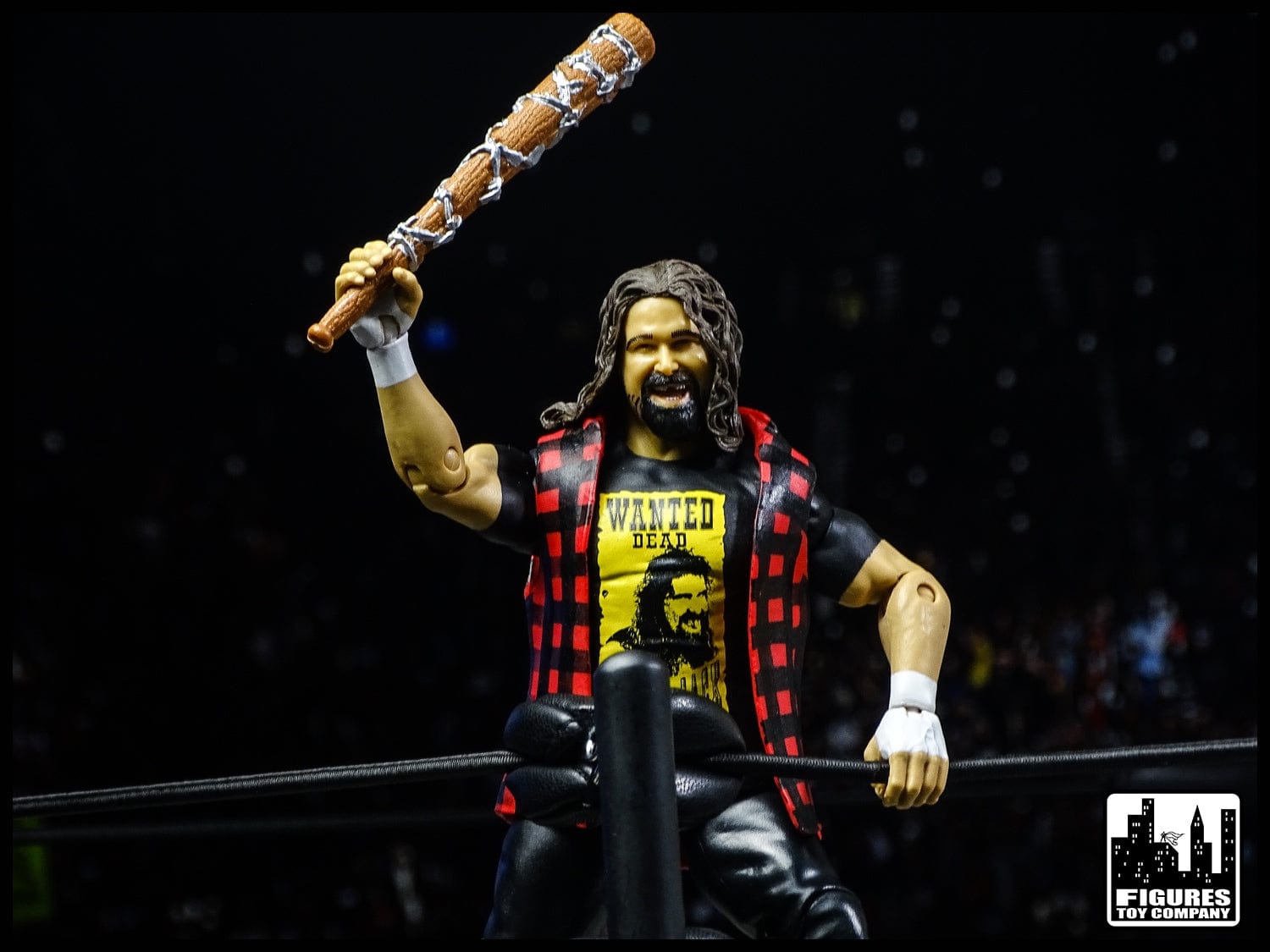The image captures a highly detailed plastic action figure of wrestler Mick Foley posed inside a toy wrestling ring. The figure features Mick Foley's iconic long brown hair and beard, with an open-mouthed smile. He is dressed in a red and black checkered flannel shirt with cutoff sleeves, over a black t-shirt displaying a yellow "Wanted Dead" poster with his face on it. The action figure's articulated arms are positioned dynamically; the right arm is grabbing hold of an elastic black rope typical of a wrestling ring, while the left hand is raised high, clutching a baseball bat wrapped in painted barbed wire. The figure's lifelike plastic skin has a smooth, almost plasticky texture. The scene is set against the backdrop of a toy boxing ring or wrestling ring, complete with metal poles and elastic ropes. In the bottom right-hand corner of the image, there is a white and black logo featuring a city skyline and the text "Figures Toy Company" emblazoned in all capital letters.